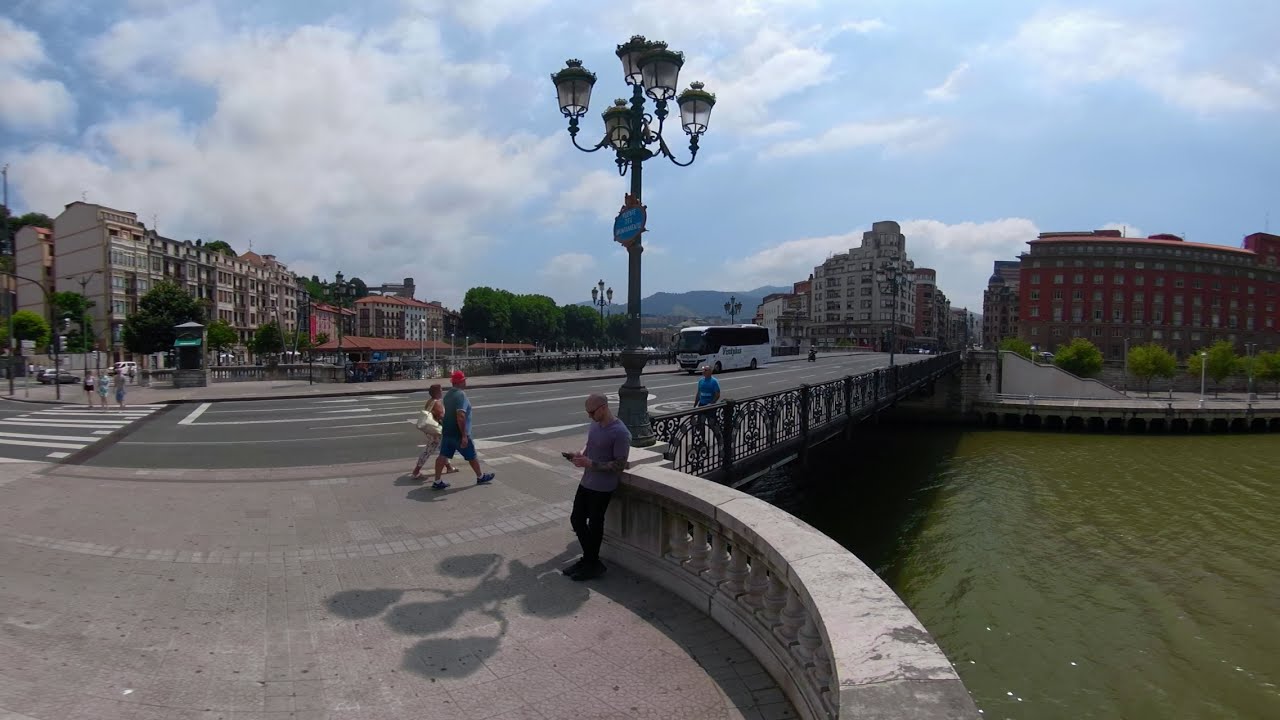The image captures a sunny day outside, featuring a scenic bridge spanning a slow-moving, greenish river. Prominently, a man in a blue t-shirt, black pants, and sunglasses with a shaved or bald head, leans against the curved stone edge of a platform near the river, engrossed in his phone. The bridge, busy with pedestrians, has people walking in various directions, including three individuals preparing to use a crosswalk. A white bus, closely followed by a motor scooter, crosses the bridge from the opposite direction. A towering light pole stands centrally, anchoring the scene framed by buildings in the distance under a sky dotted with clouds. The palette of the image is rich with diverse colors such as green, gray, and red, enhancing the lively atmosphere of this picturesque small-town setting.